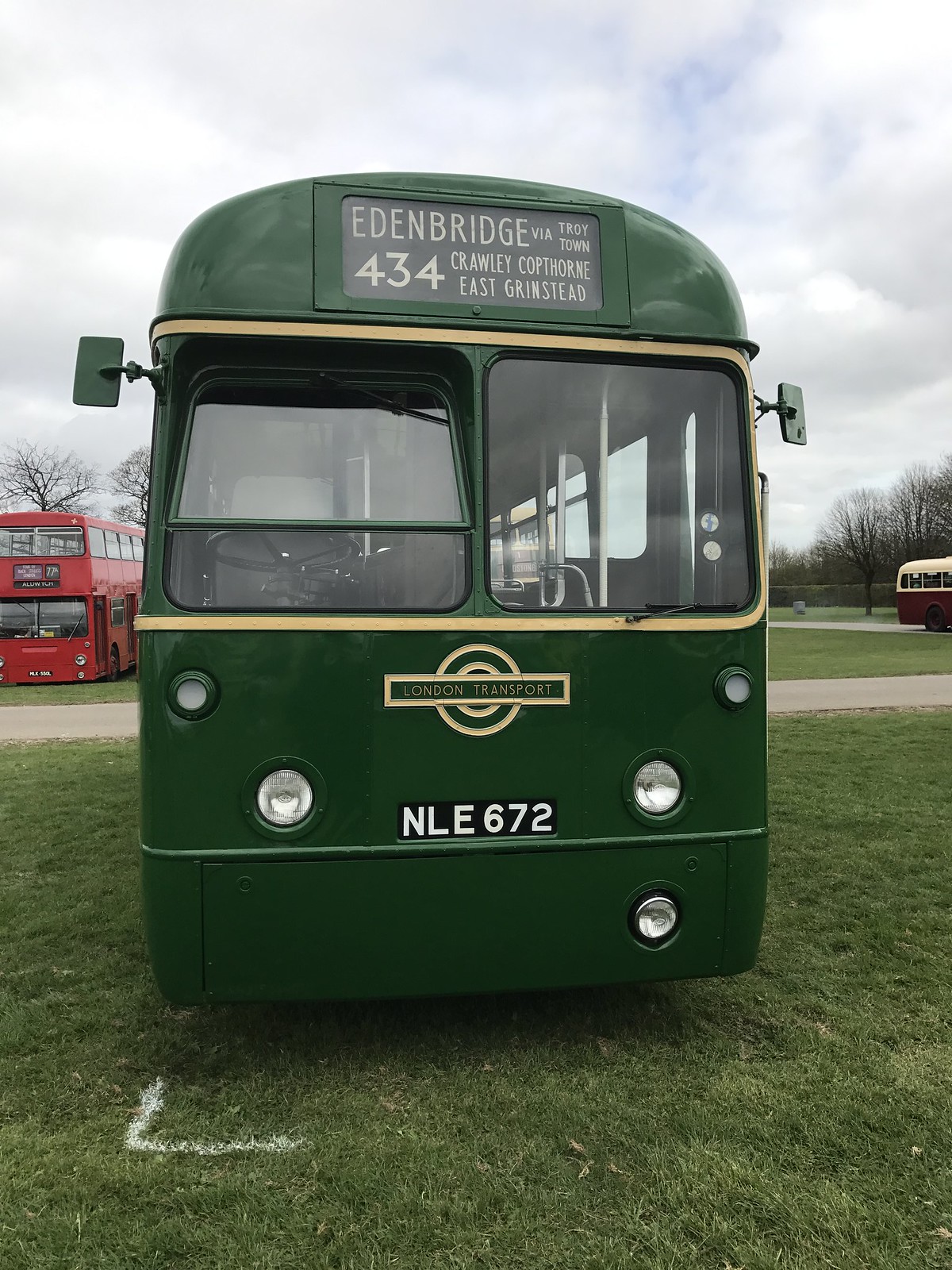This photograph showcases a dark green vintage-style London Transport bus, identified by the license plate NLE 672. The bus, parked on a grassy field, is meticulously maintained with clean windows and an overall pristine condition. The bus sports a logo with "London Transport" in pale yellow letters within a yellow rectangle on a green background, accompanied by a green and pale yellow circle. Its destination sign at the top reads "Edenbridge via Troy Town 434, Crawley, Copthorn, East Grinstead" in white letters on a black background. It is a right-hand drive vehicle, indicating its British design. The scene is set against an overcast sky, adding a moody ambiance to the setting. In the background, a red double-decker bus and a maroon and cream split-color bus are also visible, with leafless trees lining the horizon. Additionally, there's a chalk mark on the ground, suggesting designated parking for the buses.